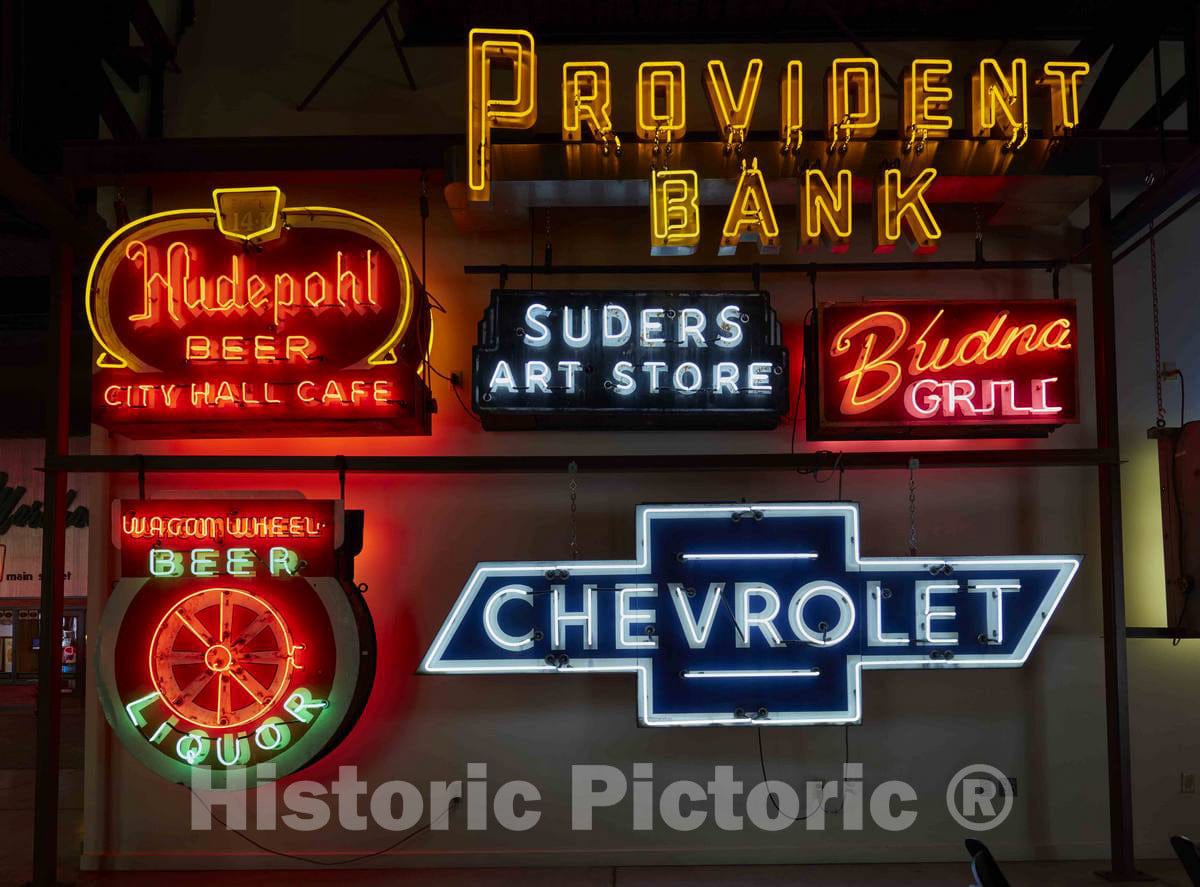This photographic image showcases a collection of six vibrant neon advertising signs against a monochromatic background. At the bottom of the image, there's a gray watermark that reads "Historic Pictoric," accompanied by a logo featuring an "R" inside a circle. The signs, arranged within a black frame, represent a variety of businesses in a spectrum of neon colors ranging from gold and blue to red, pink, green, and orange.

At the top, in gold, is a sign for "Provident Bank." Below it on the left is a sign for "Hudepohl Beer City Hall Cafe," featuring a small crown design and glowing in red and yellow. Adjacent to it, a light blue sign advertises "Suiter's Art Store." Further right is the "Budna Grill" sign, presented in pink, cursive text.

In the lower row, the leftmost sign depicts "Wagon Wheel Beer and Liquor," with a neon wagon wheel illustration and text in mint green. Finally, to the right, a blue and white "Chevrolet" sign with the iconic cross logo completes the lineup, emphasizing the nostalgic charm of these historic neon advertisements.